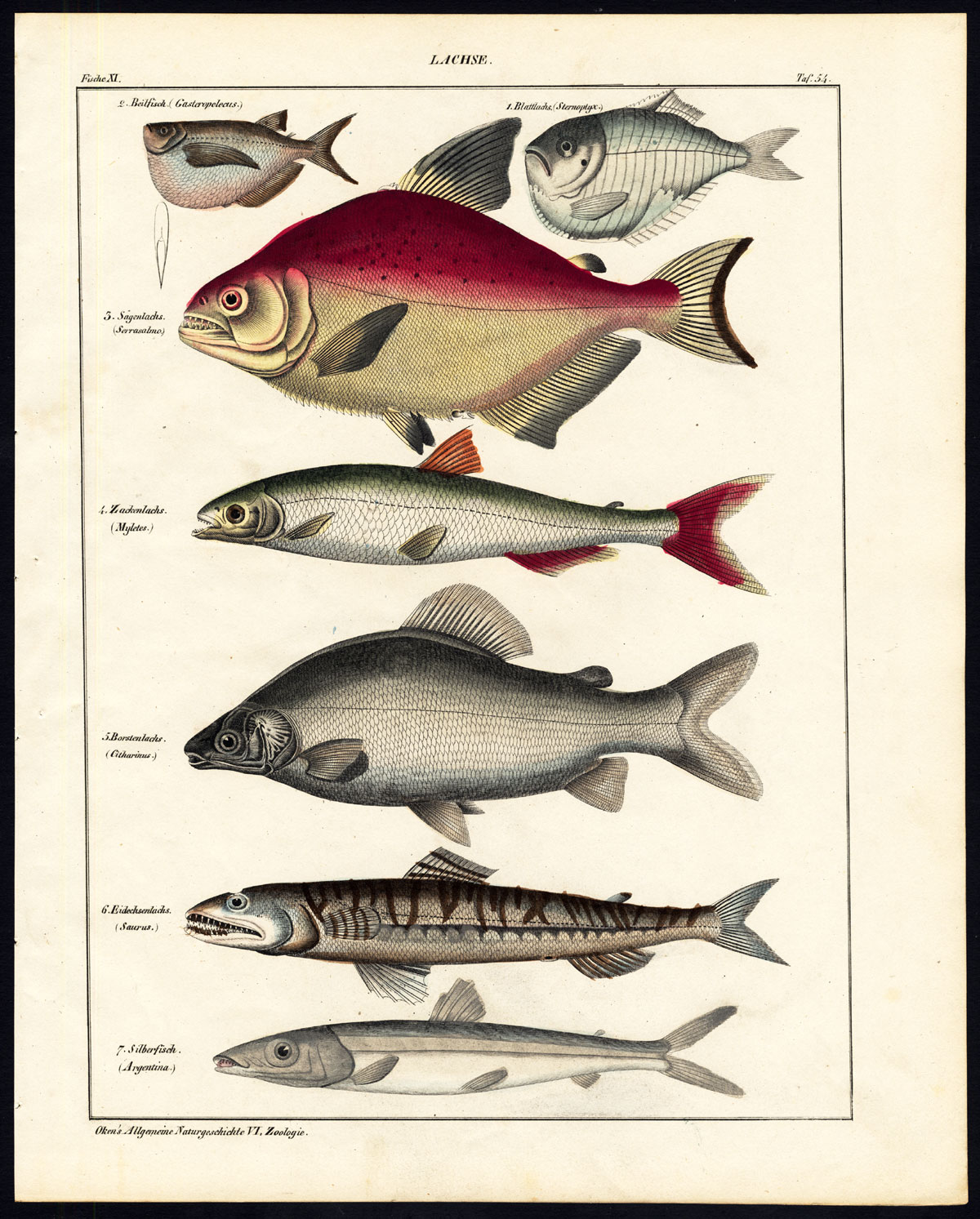This detailed photo is a framed poster depicting a variety of fish species, perfectly suited for an educational setting such as a classroom or a fishing supply store. The frame is a thin black line that elegantly borders a cream-colored background, further outlined by a thin black line that centralizes the fish illustrations. The poster features a total of seven fish, all oriented towards the left, displaying a side view.

At the top of the poster, a piece of text is partially legible, reading "L-A-C-H-S-E", while the rest of the descriptive text, presumably identifying the fish species with their Latin names, is not readable. The fish are diverse in color and size, including hues of silver, blue, red, black, yellow, brown, and white. The arrangement starts with two smaller fish at the top. Below them is the largest fish, followed by a thinner fish, a medium-sized fish, and finally, two more slim fish at the bottom.

Among the notable details, one fish at the top features vibrant red on its upper part, and another below it showcases red fins on its back. Additionally, the second fish from the bottom appears to have stripes. Each fish illustration is meticulously detailed, contributing to the academic and informative nature of the poster.